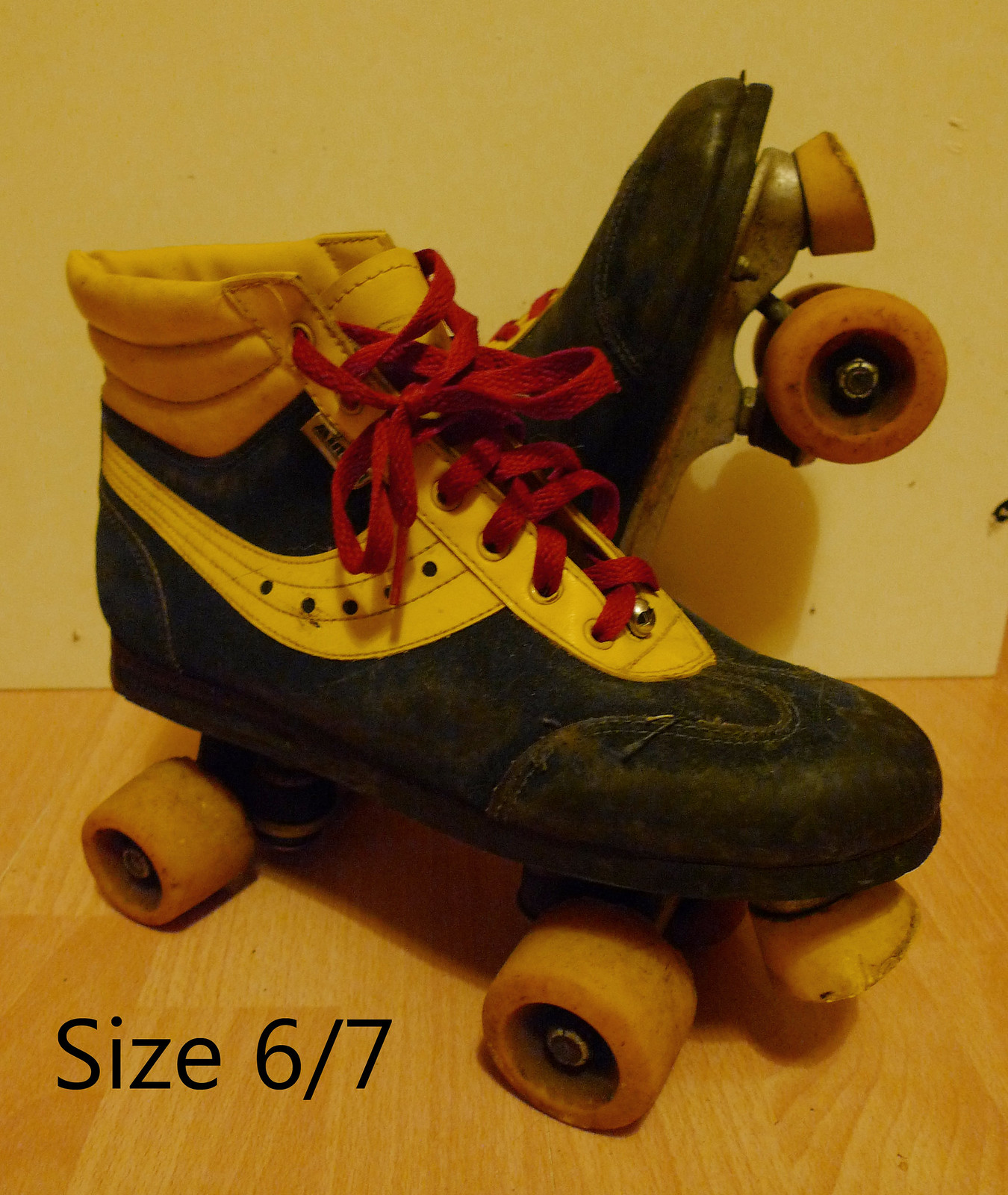An indoor color photograph features a pair of worn and antique roller skates, likely originating from the mid-50s to early 60s. The skates are crafted from leather and exhibit a well-used patina. They are predominantly black or brown with white stripes along the sides and a white band at the top, complemented by bright red laces. One of the skates is shown in a three-quarter view, detailed from the right side, while the other skate points upward toward the upper right corner, revealing its toe. The wheels are a tan color, adorned with a white front stopper, and both skates display loose threads indicating extensive use.

Set against a lighter wood floor and a pale yellowish wall, the entire image is cast in a yellow hue, giving it a vintage ambiance. Black text in the lower left-hand corner of the photo reads "size 6/7," suggesting these skates are suitable for children or teenagers. Despite their age and evident wear, these antique roller skates remain in good condition for potential purchase.